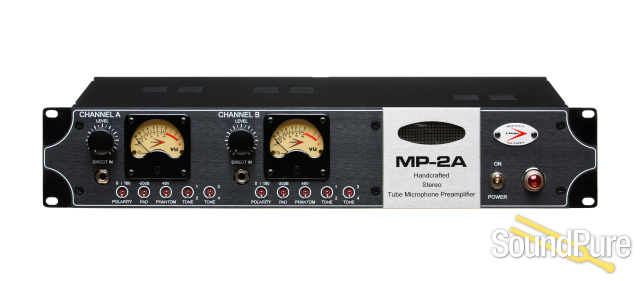The image depicts a black and dark gray rectangular preamp machine, labeled "MP-2A Handcrafted Stereo Tube Microphone Pre-amplifier." Set against a white background, it features two main channels, Channel A on the right and Channel B on the left. Each channel has a corresponding level dial surrounded by numerous dashes, a square window that contains a needle gauge transitioning from black to red to indicate levels, and a set of five plug-in ports beneath. These ports are detailed with small, likely auxiliary labels that are difficult to decipher. The front face of the machine shows additional circular mounting holes at each corner. Below the gauges, several small buttons and labels are present, though their exact descriptions are indistinct. Towards the bottom right of the preamp, there's a white oval logo with a red stripe and an on/off switch marked with the words "power," indicated by a red dot light when active.